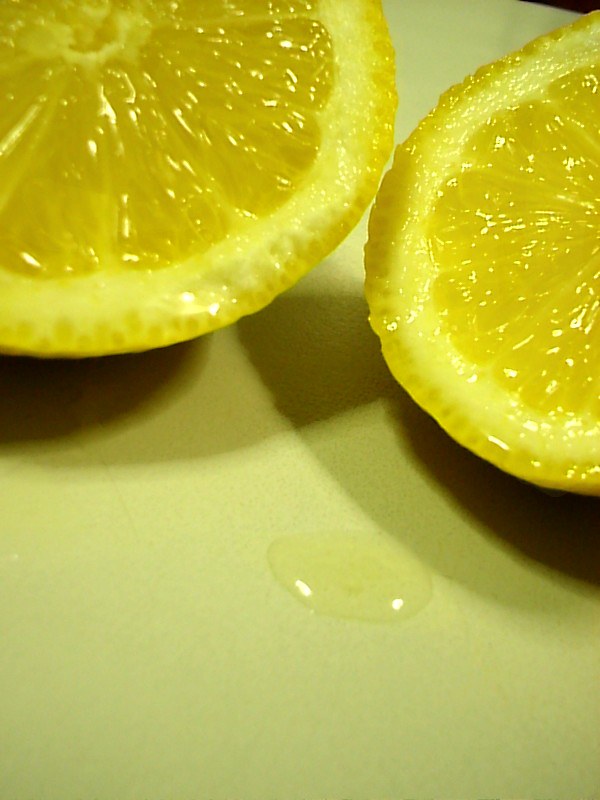The image features a lemon that has been cut in half, with each half partially visible. The lemons are placed on a yellowish-green countertop. A small pool of lemon juice can be seen on the counter towards the bottom of the picture. No seeds are visible within the lemon halves, and the background is entirely unobstructed. The countertop is bare except for the lemons, which are positioned towards the top of the image. There are no dishes or people in the frame; the lemons rest directly on the countertop.